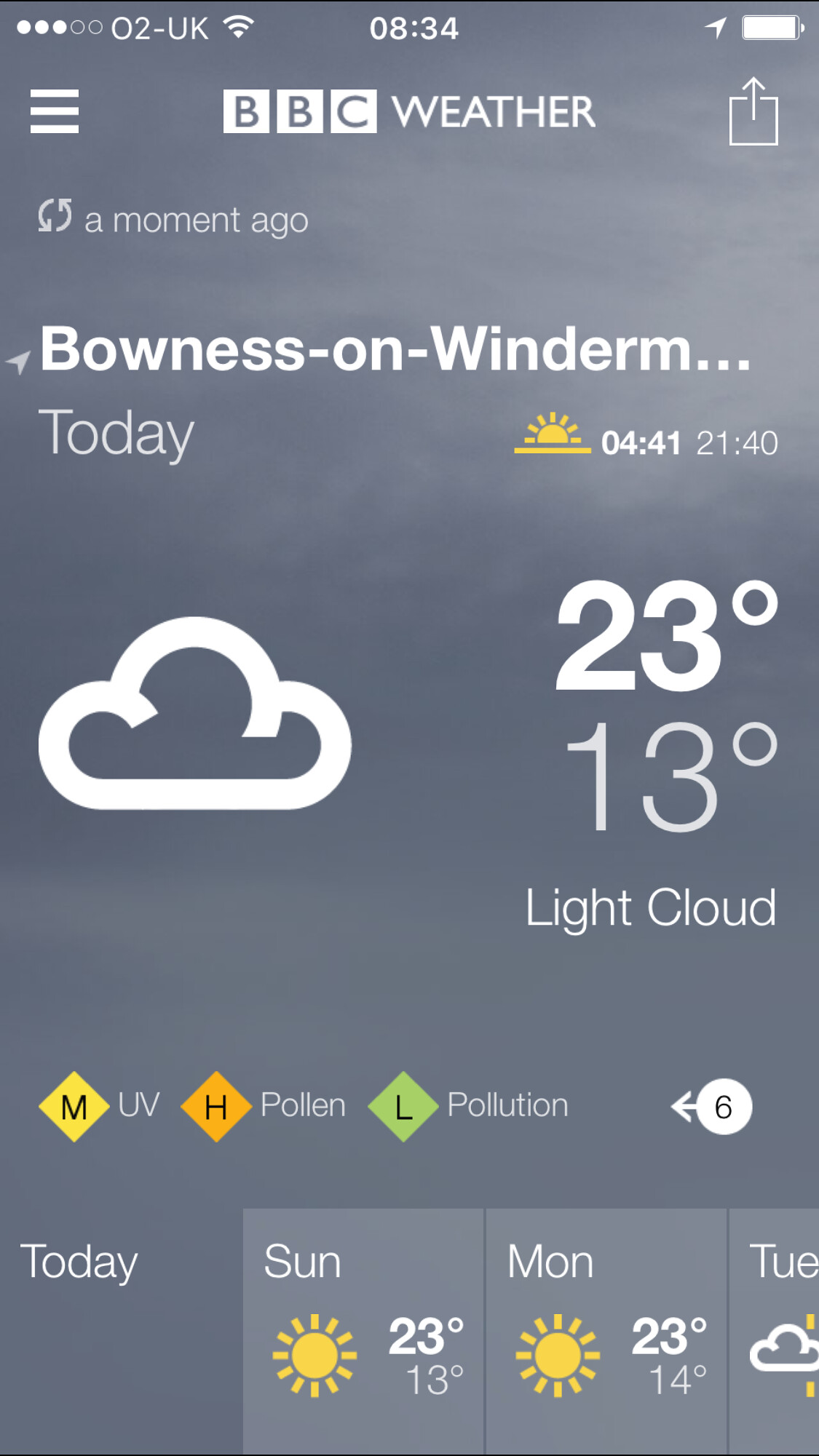This image is a detailed screenshot from an iPhone displaying the BBC Weather app. At the top, the screen shows "O2-UK" with three out of five service dots, a Wi-Fi symbol, the time "8:34", a location arrow, and a full battery icon. Just below, there is a three-line hamburger menu to the left, the "BBC Weather" title in the center, and a sharing icon to the right. The app indicates it was refreshed "a moment ago" with a refresh symbol.

In bold text, it reads "Bowness on Windermere..." with a sun setting icon, and times "4:41" and "21:40" next to it. Below, there's a cloud icon showing "23°C" above "13°C" with a description "Light cloud". Further down, there are three rectangular indicators: a yellow MUV symbol, an orange "H" for pollen, and a green "L" for pollution. A circle with the number "6" and a left arrow (representing a downtrend) is also visible. 

At the bottom of the app display, it reads "Today", followed by weather forecasts for Sunday, Monday, and Tuesday with associated sun icons and temperatures. The information for Tuesday is partially cut off.